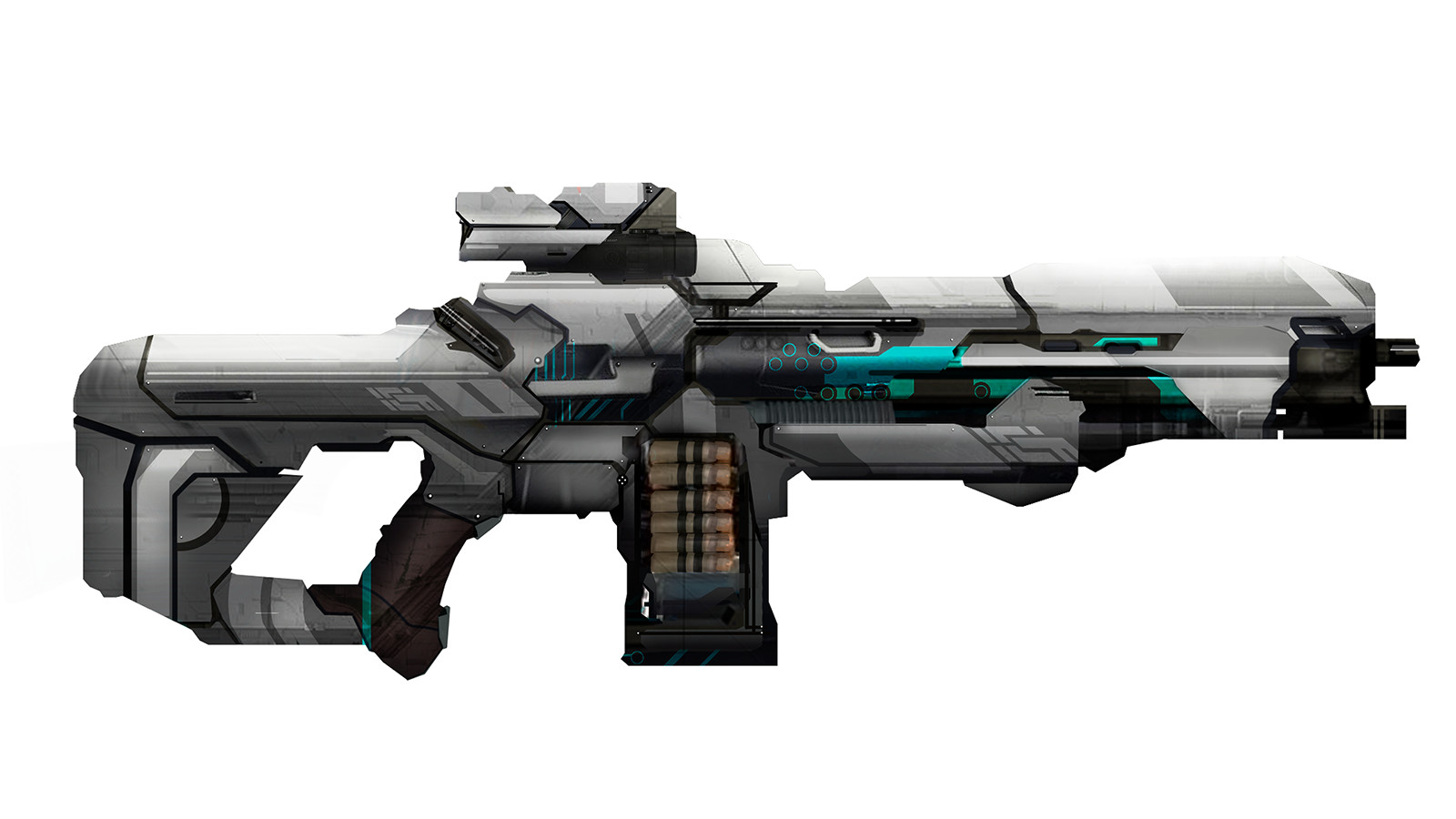The image features a highly detailed, computer-generated depiction of a futuristic assault rifle set against a white background, resembling a photo taken in a lightbox. The rifle is distinctly high-tech and diverges significantly from conventional designs. Its barrel is short, only a few inches of which are visible, protruding from a rectangular, chunky housing that gives the gun a robust and enclosed appearance. The weapon's grip, resembling those commonly found in video games, is connected to a square and thick stock, enhancing its futuristic aesthetic.

A notable feature of the gun is its depiction of advanced technology, with a laser sight mounted at the top and subtle teal and green accents, possibly indicating lights or additional tech elements. The rifle is primarily composed of varying shades of gray, from light to dark, and appears to be constructed of plastic rather than metal, emphasizing its modernistic design. Additionally, the rifle is equipped with a large magazine loaded with substantial cartridges, featuring brass tips and light green casings, suggesting powerful ammunition. The overall composition and details suggest that this rifle is designed more as a conceptual or fictional weapon, likely intended for a video game setting.